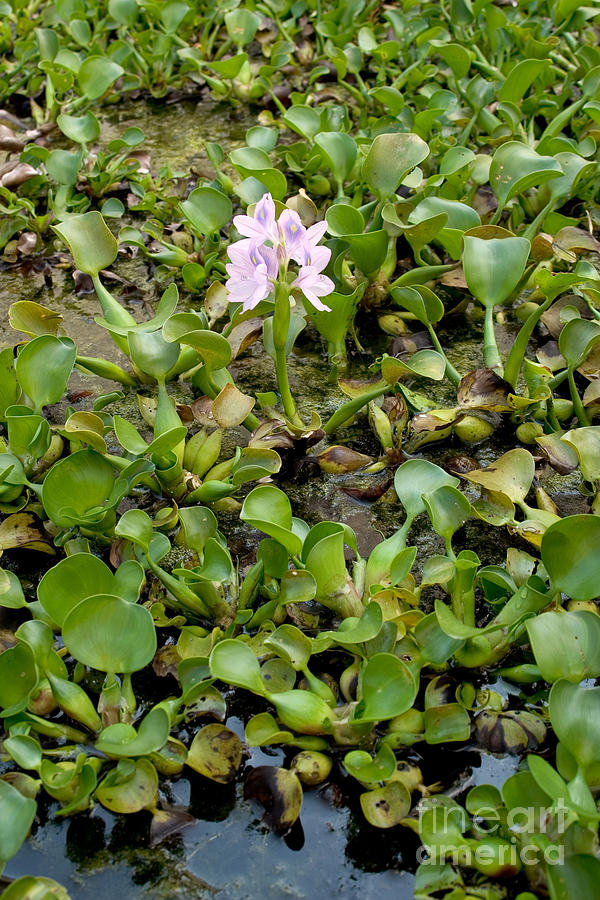The image depicts an outdoor scene on a cloudy day, featuring a dense array of small plants with thick, circular leaves, many of which are growing in standing water that occupies about a fourth of the vertical frame. Most of the leaves extend above the water, with some appearing dirty with black spots. Among these leaves, one stands out as being half-covered in soil or soot. The plants give an impression of increasing dryness as they grow higher, maintaining their circular leaves. Notably, in the center of this green expanse, a unique plant with a tall green stem and delicate, light pink to purple flowers blooms, contrasting against the predominantly leaf-covered plants. This flowering plant adds diversity with its two or three distinct blossoms. In the bottom right corner, the text "fine art America" is inscribed, with "fine" appearing numbered and "art" and "America" in all lowercase letters.